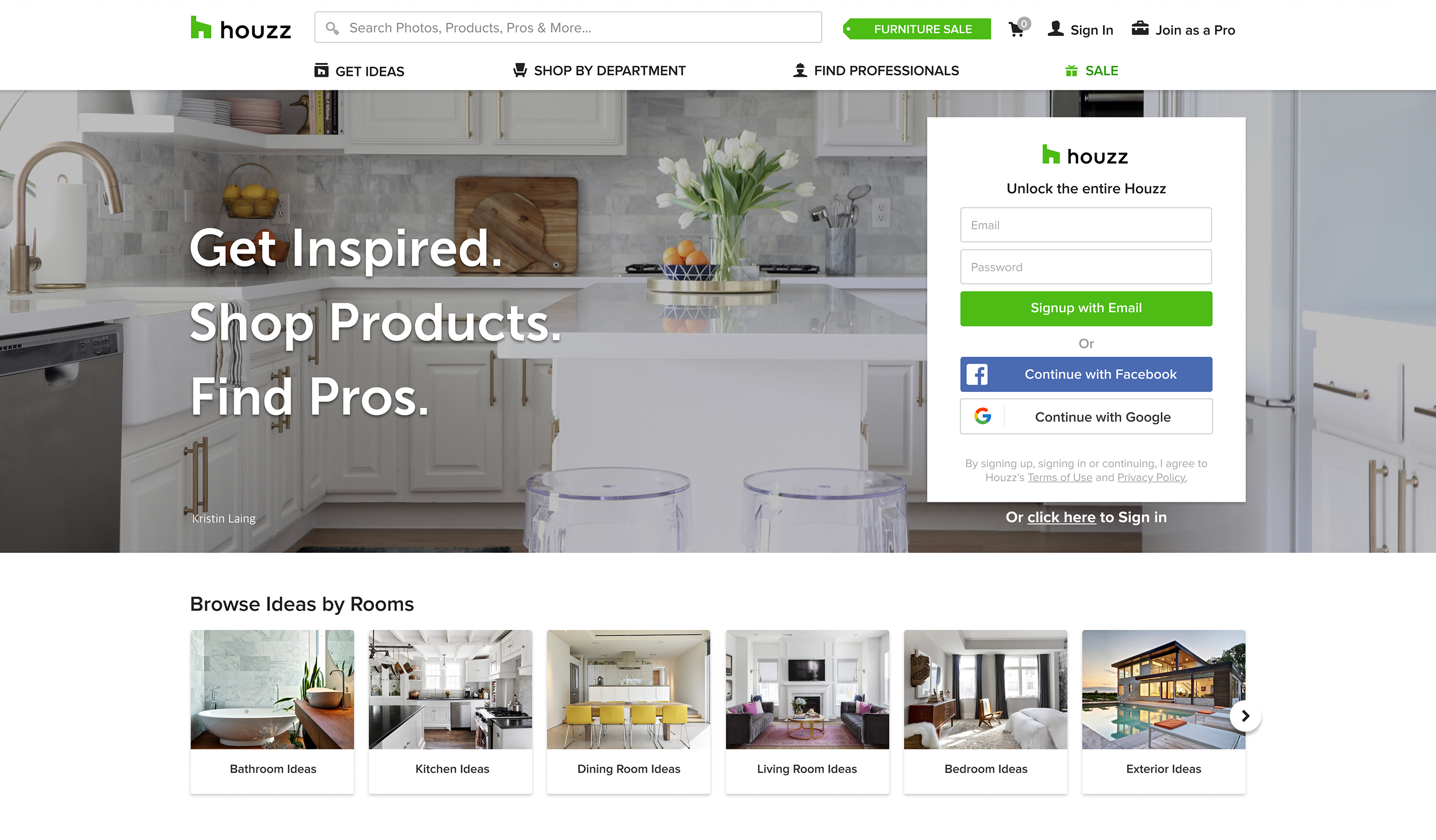This image displays a screenshot of the Houzz website's homepage, showcasing its user-friendly interface and various features. At the top of the page, the well-known green Houzz logo, spelled "H-O-U-Z-Z," is prominently displayed. Directly beside the logo is a search bar where users can look for photos, products, professionals, and more. A green banner announcing a "Furniture Sale" is adjacent to the search bar, along with a shopping cart icon that currently shows no items.

Users are given options to "Sign In" or "Join as a Pro" at the top-right corner. 

Beneath the header, there is a navigation menu with four main categories: "Get Ideas," "Shop by Department," "Find Professionals," and "Sale," with the "Sale" tab highlighted in green. Below this menu, a visually appealing, well-designed kitchen is featured as the background image. Superimposed on the left side of this picture are the prompts: "Get Inspired," "Shop Products," and "Find Pros."

Hovering above the kitchen image is a sign-up box inviting users to "Unlock the Entire Houzz." This box contains fields to input an email and password, along with options to sign up via email or continue using Facebook or Google. A note below this invites users to "click here to sign in," which is underlined for emphasis.

Further down, the website showcases categories to browse ideas by rooms with six images, each representing different parts of a house. These categories include "Bathroom Ideas," "Kitchen Ideas," "Dining Room Ideas," "Living Room Ideas," "Bedroom Ideas," and "Exterior Ideas," arranged from left to right. An arrow to the left suggests there are additional categories to explore.